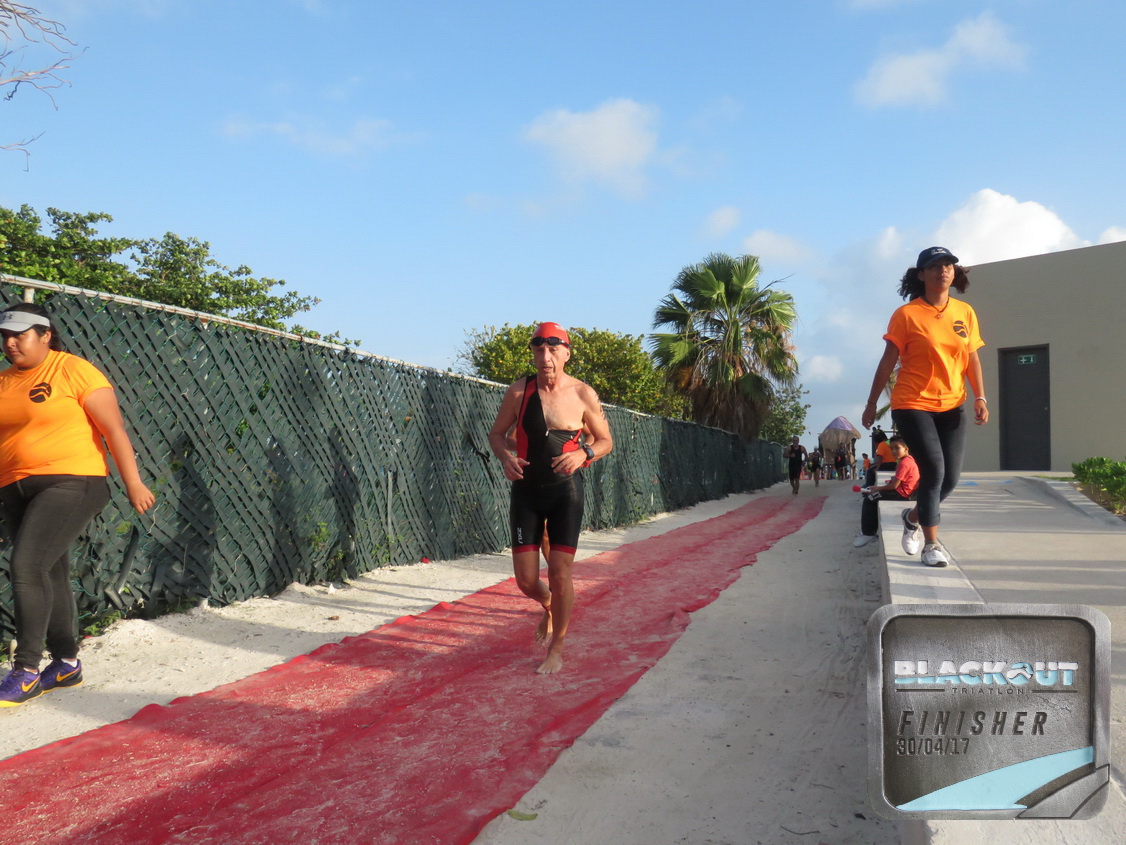The photograph captures a vibrant finish line for a marathon or triathlon, featuring a long red carpet semi-covered in sand and flanked by white grainy sand. Dominating the left side is a tall chain-link fence with a green tarp. In the foreground, a barefoot elderly man, appearing to be in his 70s and wearing a swim cap and goggles on his forehead along with a wetsuit, runs energetically along the red carpet towards the finish line. On the left side of the image, a person with purple shoes adorned with yellow check marks, clad in black tight pants, and a yellow short-sleeved shirt with a black circle logo, watches the race, sporting a green visor. To the right of the red carpet, a woman steps onto a concrete walkway; she wears white shoes, black short pants, and a yellow short-sleeved shirt with a black circle logo. In the bottom right corner of the image, text imposed over the photo reads, "Blackout Triathlon Finisher 30/04/17," marking the event's completion date. More runners can be seen approaching in the distance, adding to the scene's energetic atmosphere.